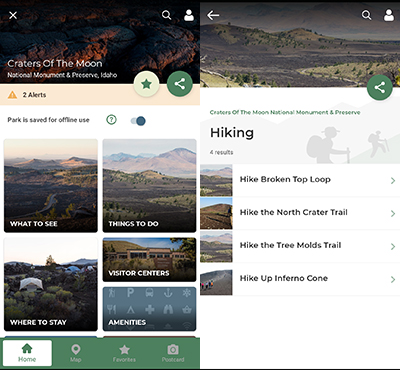The image appears to be a screenshot from a website or an app dedicated to a hiking company, specifically showcasing Craters of the Moon National Monument and Preserve in Idaho. The layout includes multiple sections with various photographs and informative titles.

In the top left corner, there is a captivating photograph resembling a cave, accompanied by the text "Craters of the Moon National Monument and Preserve, Idaho." Adjacent to this, on the right, is an expansive view of mountains and open land.

Below these main images, there are several sections labeled with informative headings: "What to See," "Things to Do," "Visitor Centers," "Amenities," and "Where to Stay." Each section is illustrated with relevant pictures featuring landscapes, hills, buildings, and visitor centers.

To the far right, a section titled "Hiking" is displayed along with a list of various hiking trails:
- "Hike Broken Top Loop" accompanied by a representative image.
- "Hike the North Crater Trail" with a picture of a scenic hill.
- "Hike the Tree Molds Trail" featuring imagery of land and hills.
- "Hike Up Inferno Cone" displaying hikers ascending a brown hill.

At the bottom left of the screen, there is a home button icon, depicted as a small white house, which appears to be selected. To its right, there are additional navigational options labeled "Map," "Favorites," and a camera symbol, likely for accessing a photo gallery or taking pictures.

Overall, the screenshot provides a detailed and organized overview of Craters of the Moon National Monument and Preserve, highlighting key attractions and hiking opportunities.